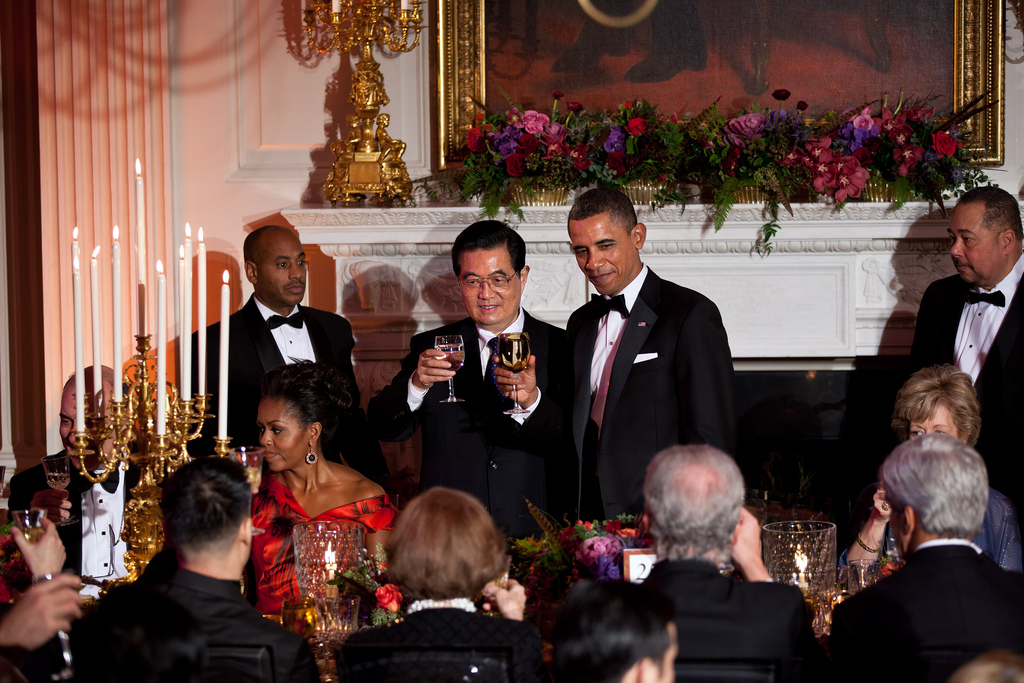In this photograph, President Barack Obama is seen standing at a state function, impeccably dressed in a tuxedo. He is holding a gold goblet, participating in a toast. Three men, also in tuxedos, stand next to him. The man immediately to his left is wearing glasses and holding a clear glass. 

The background is a scene of elegance and grandeur, with an elaborate white carved fireplace adorned with a gold candelabra and another gold object on the mantle. A luxurious arrangement of plum, purple, burgundy, pink, and red flowers with green leaves adds to the opulence. A gold-leaf painting with a burgundy background hangs above the fireplace, enhancing the sophisticated atmosphere.

Guests are seated at tables, most dressed in black attire, except for an older woman in a navy dress. Michelle Obama is also present, elegantly dressed in a red and black gown with dark-colored earrings. The room is illuminated by white tapered candles in the candelabra, which adds a warm glow to the scene, signifying a moment of celebration and refinement.